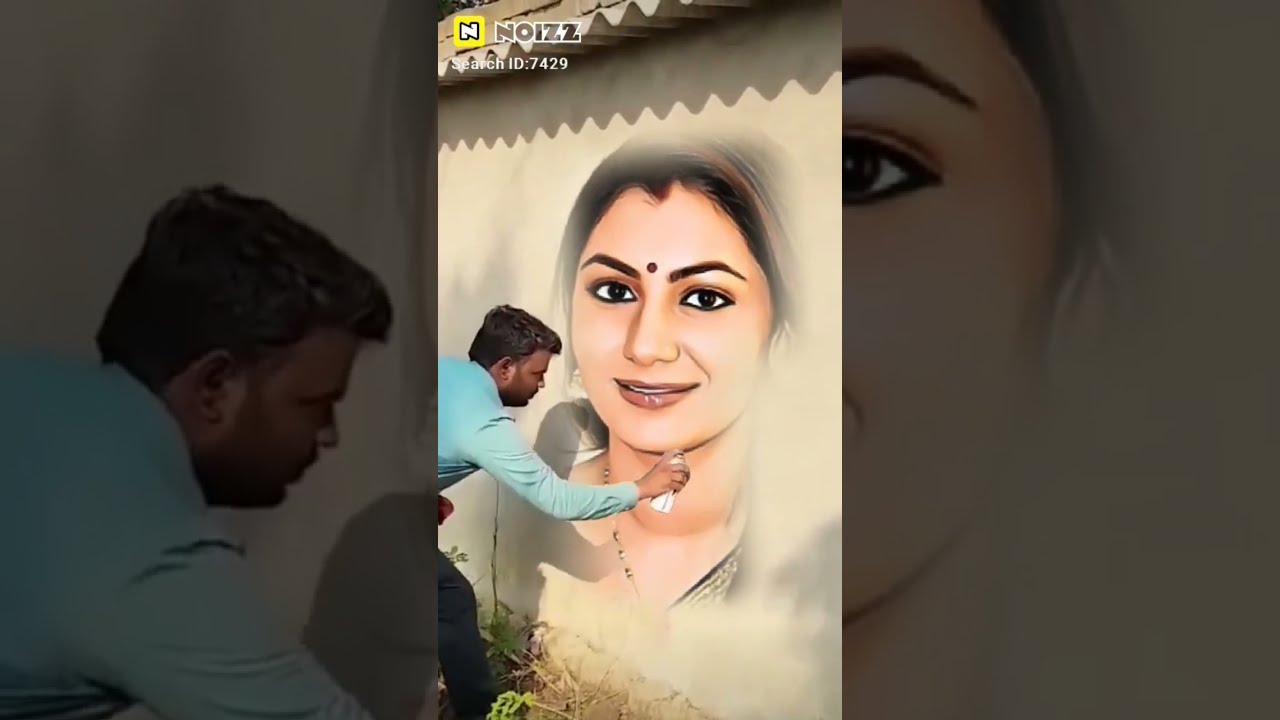The image depicts a close-up view of a man with dark brown skin and dark hair, standing near the left-hand side of a cream-colored wall outside, spray painting a portrait of a lady. He is wearing a long-sleeved blue shirt and dark pants and is holding a white spray bottle in his right hand near the chin area of the portrait. The middle panel shows the man painting a detailed image of an Indian lady with black hair, a red dot on her forehead, brown eyes, dark brown eyebrows, and a red mouth. She appears lifelike with glistening lips and a subtle smile, and is wearing a gold shirt. This middle scene is flanked by two side panels that fragment and zoom in on the man's head and the woman's face. The scene is framed under a short awning on top of the building exterior. The image includes a header with "NOISE" in a yellow square with a white 'N' bordered in black, with "search ID 7429" as a watermark, suggesting it may be from a TikTok or Instagram reel due to its smartphone aspect ratio.